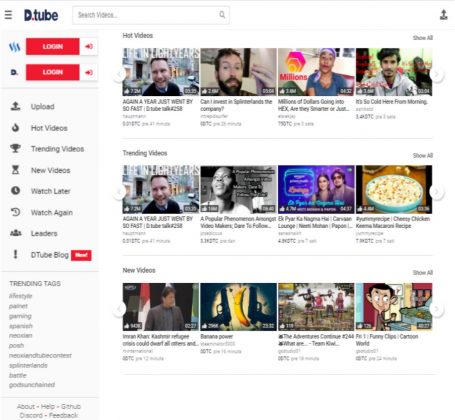This image is a detailed screenshot of the D-Tube website, an emerging video-sharing platform. At the very top of the site is the D-Tube logo, prominently displayed on the left. Adjacent to the logo, on the right side, is a search bar with placeholder text reading, "Search videos." 

On the left side, there are login buttons, providing two options for users to log in, likely through different methods. Directly below the search bar, you’ll find navigation links for various sections of the site: "Upload," "Hot Videos," "Trending," "New Videos," "Watch Later," "Leaders," and "D-Tube Blog."

Below these options, there's a section labeled "Trending Tags," which includes a variety of tags like #Lifestyle, #Gaming, #New, #Palnet, #Crypto, #DTube, #Technology, #SCT, #Marlands, and #Neo-Xen.

The main content of the page is divided into three sections: "Hot Videos," "Trending Videos," and "New Videos." 

In the "Hot Videos" section, a few highlighted videos include:
1. "Again a year just went by" by D-Tube with 185 views, uploaded 12 hours ago.
2. "Can I Invest in Splinterlands the Company?" by Andy with 175 views, uploaded 18 hours ago.
3. "Millions of Dollars Going into HEX. Are They Smarter or Just Crazy?" by HEXologist with 720 views, uploaded two days ago.
4. "It's Cold Here! Free from Morning Even" by German with 118 views, uploaded three days ago.

The "Trending Videos" section features:
1. "Popular Phenomenon Again: Among Us is a Bad Idea" by Emily with 145 views, uploaded one day ago.
2. "D-Tube Blog" by Nag Ham with 332 views, uploaded two days ago.
3. "Cry Mini Pretz Chicken with Prawn" with 80 views, uploaded four hours ago.

The "New Videos" section showcases the latest uploads, complete with thumbnails.

Finally, the footer of the site includes links to “About,” “Help,” “GitHub,” “Discord,” and “Feedback.” The overall layout is straightforward and user-friendly, bearing a resemblance to YouTube's interface.